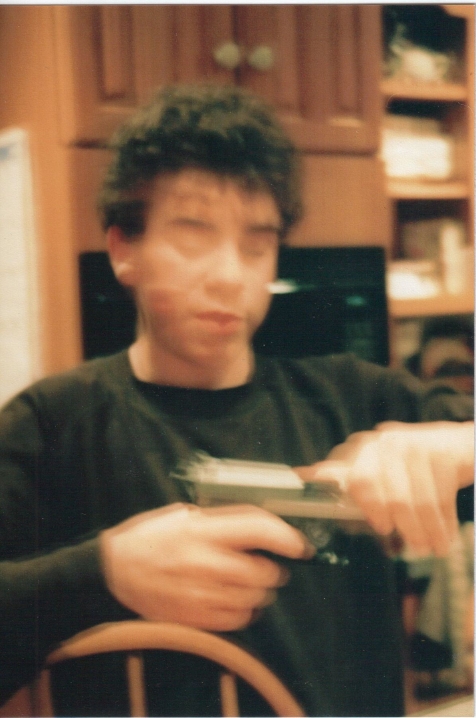This is an extremely blurry, close-up color photo of a very young man standing in a kitchen. The kitchen features brown cabinets, with overhead cabinets above what appears to be a black microwave or oven. To the right, there are open brown wood shelves resembling cabinets without doors, possibly holding stacks of white dishes or plates. In the background, there's the outline of a doorway. The young man, who has short curly brown hair and pale beige skin, is wearing a dark-colored, long-sleeved shirt. He is holding a silver and black revolver, with his right hand gripping the handle and resting on a light brown oak wooden chair, while his left hand holds the muzzle.